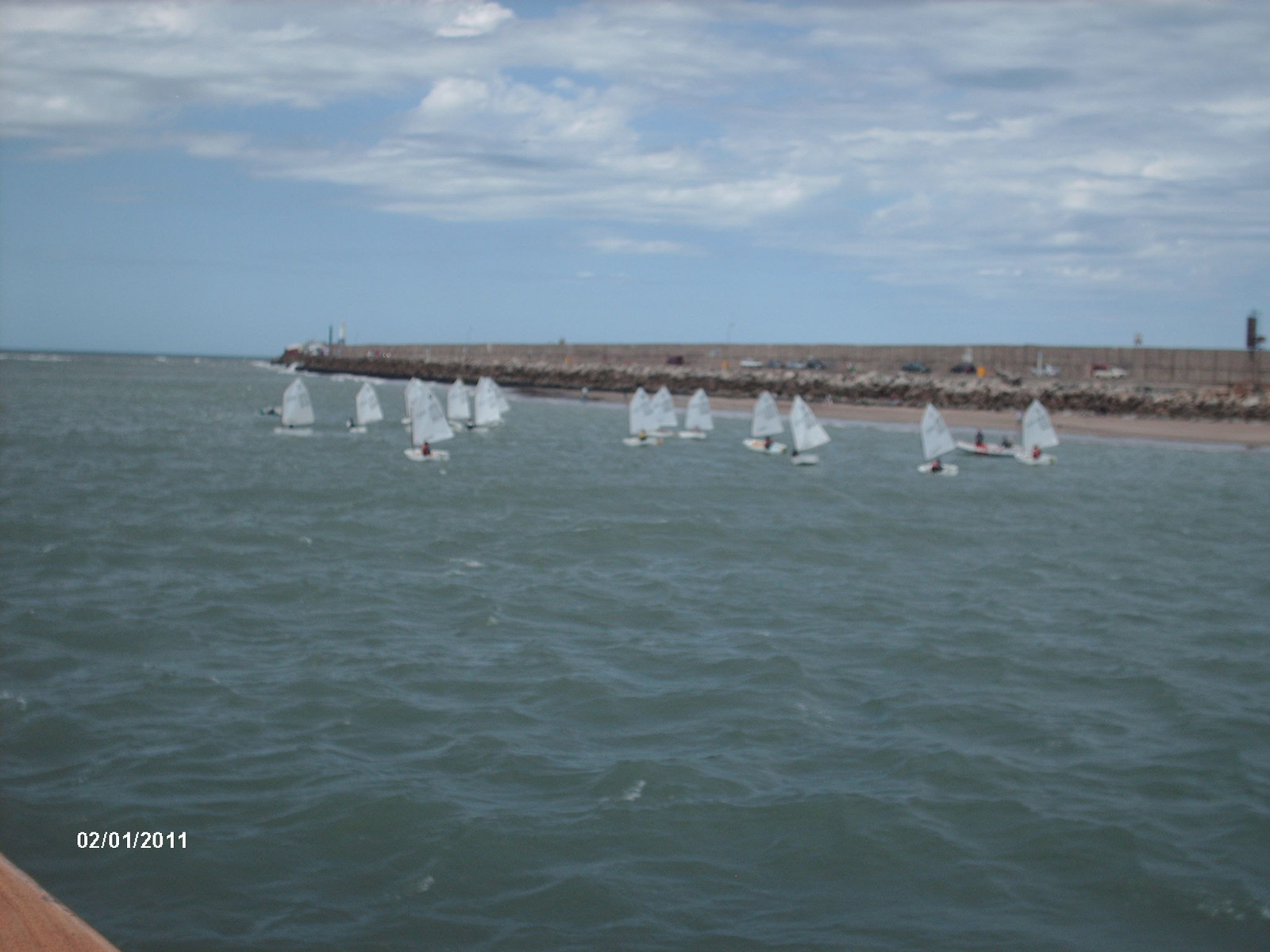This image, dated February 1st, 2011, captures a slightly blurred scene of a cold and cloudy day at the ocean. Taken from a boat — a bit of which is visible in the corner — this photo showcases about 20 small sailboats, each with a single white sail, seemingly engaged in a race. The water appears gray and deep, reflecting the overcast sky. In the background, a jetty or break wall stretches into the horizon, beyond which some vehicles can be discerned. The boats, approximately 50 feet from the shore, hint at a beachfront scene, possibly used for training or practice in sailing. Despite the low contrast and drab coloring suggesting it might be an old, perhaps scanned photograph, the atmosphere remains bright amidst the predominantly cloudy sky.